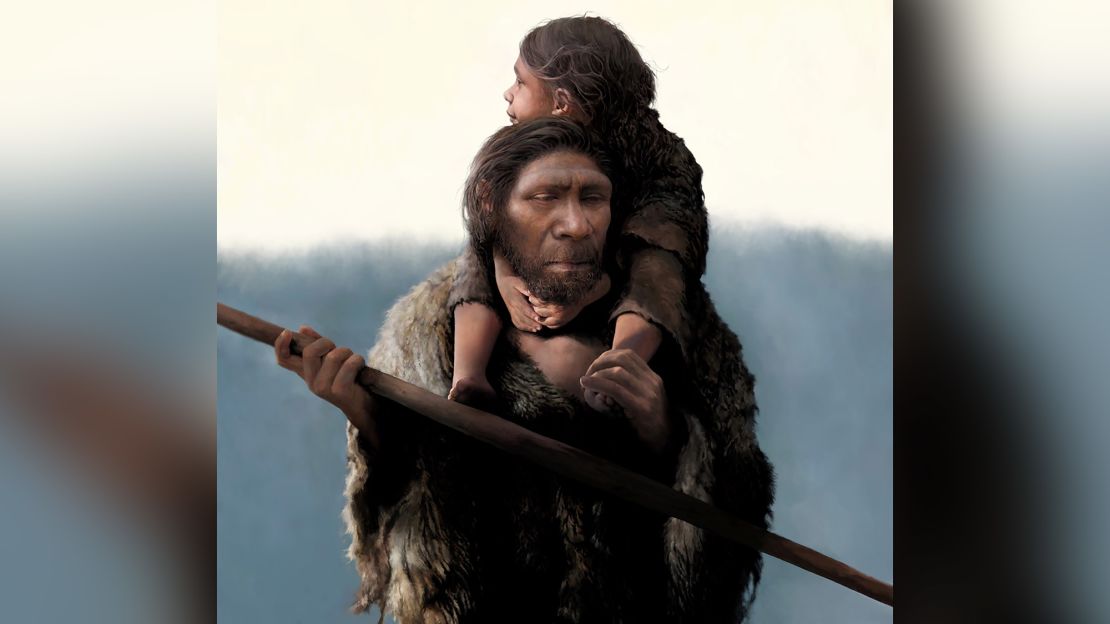In this digital rendering of a Neanderthal, the scene is set outdoors with a light, cloudy sky in the background and darker, blurred edges framing the image to focus attention on the central figures. The main character, a tall Neanderthal man, has distinctive facial features, including a wide nose and a short forehead, further characterized by his longer brown hair pulled back and a beard. He wears a fur coat and holds a long rod or staff in his right hand. Seated on his shoulders is a child also dressed in furs, whose feet rest around the man's neck. The man grips the child's left foot with his left hand while the child clasps their hands together near their chin. The man gazes downward toward the lower right corner of the image, while the child looks away, towards the upper left. Behind them, the backdrop hints at a mountainous region, contributing to the ancient atmospheric setting.